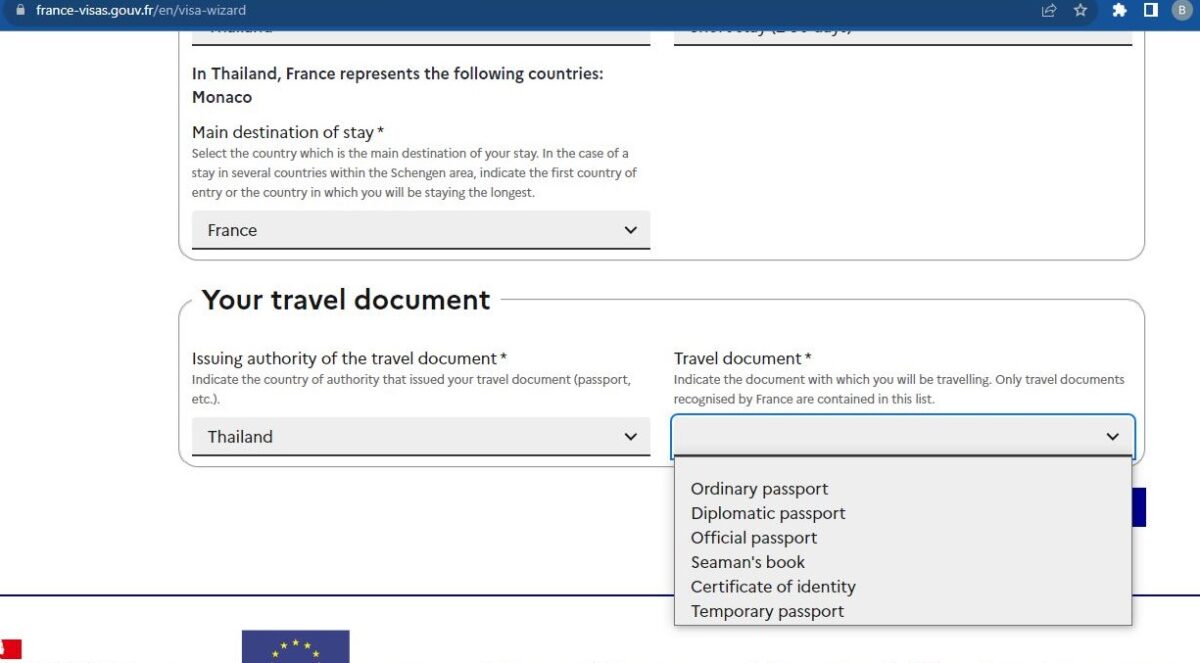The image displays a detailed screenshot of a website, specifically the France Visa Wizard page. 

At the top of the screenshot is a blue address bar with white text that reads "france-visas.gov.fr/en/visa-wizard." To the left of this text, there is a lock symbol indicating a secure connection. On the extreme right of the address bar, several icons are visible, including a sharing symbol, a star, a puzzle piece, a white square, and a grey circle with a "B" inside it.

Beneath the address bar, the background of the website is predominantly white. Centrally aligned on this section is a black-bordered box containing text. The text inside this box reads: "In Thailand, France represents the following countries’ consulate." Below this, another line of text states: "Main destination of stay: Select the country which is the main destination of your stay. In the case of a stay in several countries within the Schengen area, indicate the country of entry in which you will be staying the longest."

Following this instruction, there is a grey drop-down box labeled "France." Below, another section titled "Your travel document" is enclosed within a thin black border. Within this section, to the left of a text box, the label reads: "Issuing authority of the travel document," followed by an asterisk. Beneath this label, in slightly smaller text, it says: "Indicate the country of the authority that issued your travel document (passport, etc.)." A grey drop-down box with the label "Thailand" is positioned below.

To the right of the image, another section headed "Travel document" advises: "Indicate the document with which you'll be travelling. Only travel documents recognized by France are contained in the list." This instruction is followed by an empty grey drop-down box with the label "Select." Below this drop-down are various types of travel documents listed as options, including: "ordinary passport, diplomatic passport, official passport, seaman's book, certificate of identity, or temporary passport."

At the bottom of the visible portion of the screenshot, there is a black-bordered box encasing more text. On the left side of the image, partially cut off, is the EU flag.